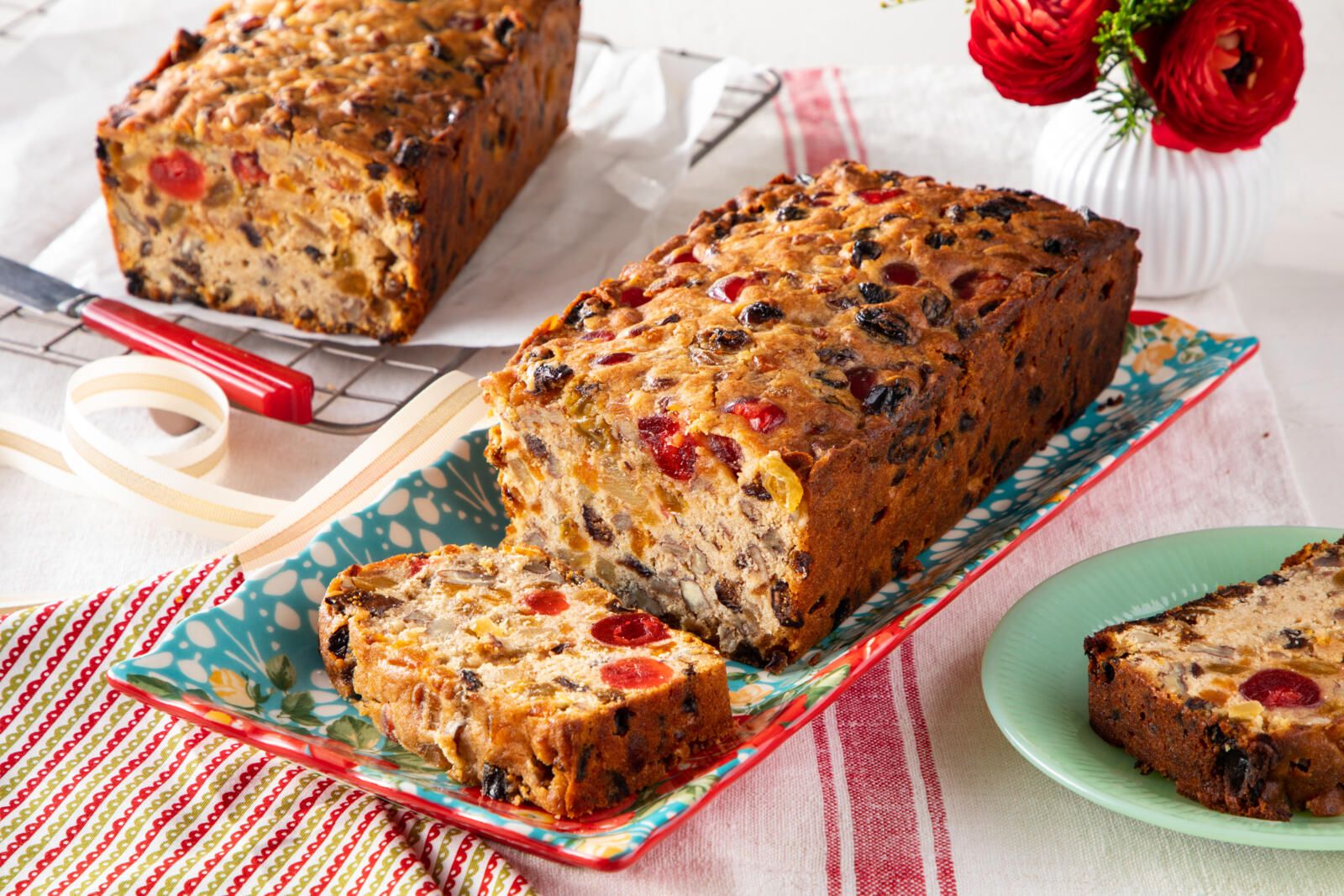This contemporary photograph, likely from a couple of decades ago, beautifully captures a holiday-themed setting centered around fruitcake, a traditional festive treat in the United States. The scene is laid out on a white tablecloth adorned with a tea towel featuring alternating red and green stripes, evoking Christmassy colors.

In the middle of the image, a rectangular serving dish, decorated in vibrant hues of aqua, red, and yellow, holds an entire loaf of fruitcake. One slice has been cut from the loaf and positioned on its side, revealing the dense, intricate mixture of cherries, nuts, and various dried fruits inside. This sliced loaf is accompanied by a distinct red-handled knife positioned on the left. Next to it, another piece of fruitcake sits on a green plate, capturing the viewer's attention.

To the upper left, atop a wire rack, lies another loaf of fruitcake, resting on a napkin. A small white vase containing two striking red flowers, adding a pop of color to the scene, can be seen in the upper right corner of the photograph. The image is clear, and the composition thoughtfully combines the rich textures and colors of the fruitcakes with festive decorations, emphasizing the warmth and tradition of the holiday season.